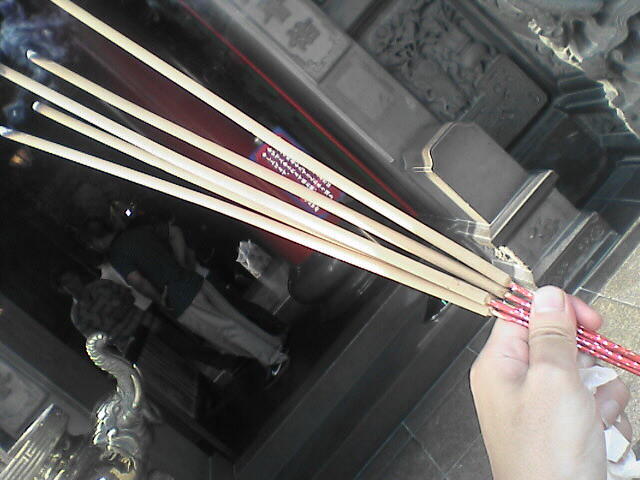A close-up image depicts a fair-skinned hand, possibly female, with long nails, grasping five incense sticks or joss sticks by the red-speckled handles. The sticks, which are thin and extend diagonally from the bottom right to the top left corner of the image, appear to be made of natural beige wood and show burn marks at their tips. The hand is in front of an ornate stone building adorned with Asian writing and featuring a decorative elephant structure on the left. The building has a gray exterior with intricate carvings and a prominent red feature visible through the entrance. Inside the slightly darkened doorway stand two men, one visibly wearing a dark shirt with tan pants and the other with his hands on his hips. Despite the busy background, the focus remains on the bright red-handled incense sticks held firmly by the hand.